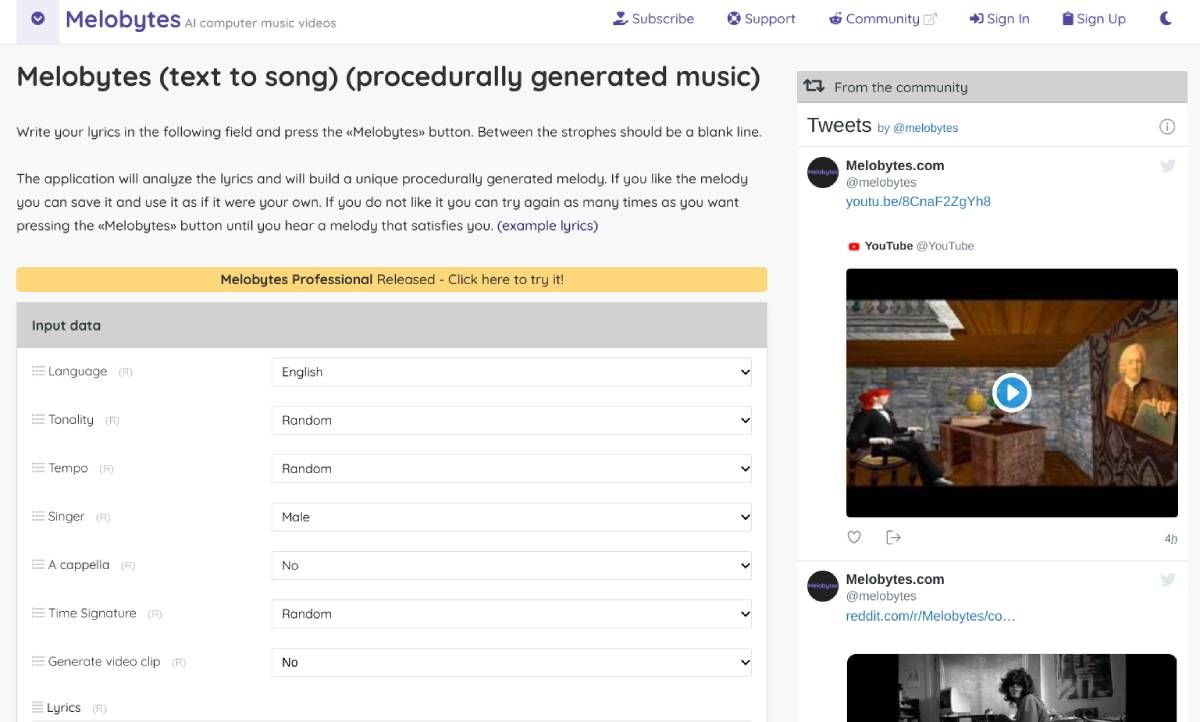**Detailed Caption:**

In the image, we see a screenshot of the interface for "Mellow Bites AI Computer Music Videos," prominently displayed in the upper left-hand corner. In the upper right-hand corner, there are several navigation tabs labeled: "Subscribe," "Support," "Community," "Sign In," and "Sign Up," accompanied by a moon icon. 

Beneath this header, there's a prominent title that reads, "Mellow Bites (Text to Song) - Procedurally Generated Music." Below this title is an instructional segment encouraging users to write their lyrics in the provided field and press the "Mellow Bites" button. This section explains that the application will analyze the submitted lyrics and generate a unique melody based on them. Users can keep trying until they find a melody that they like, as many times as they wish. If satisfied, the melody can be saved and used as if it were their own creation.

The image also displays a sample prompt that reads, "Mellow Bites Professional Released. Click here to try it." Additionally, there is an input data section featuring multiple drop-down menus for customizing the music generation process. These options include language, tonality, tempo, singer, a cappella (yes/no), time signature, and an option to generate a video clip. There is also a large text box designated for entering the lyrics.